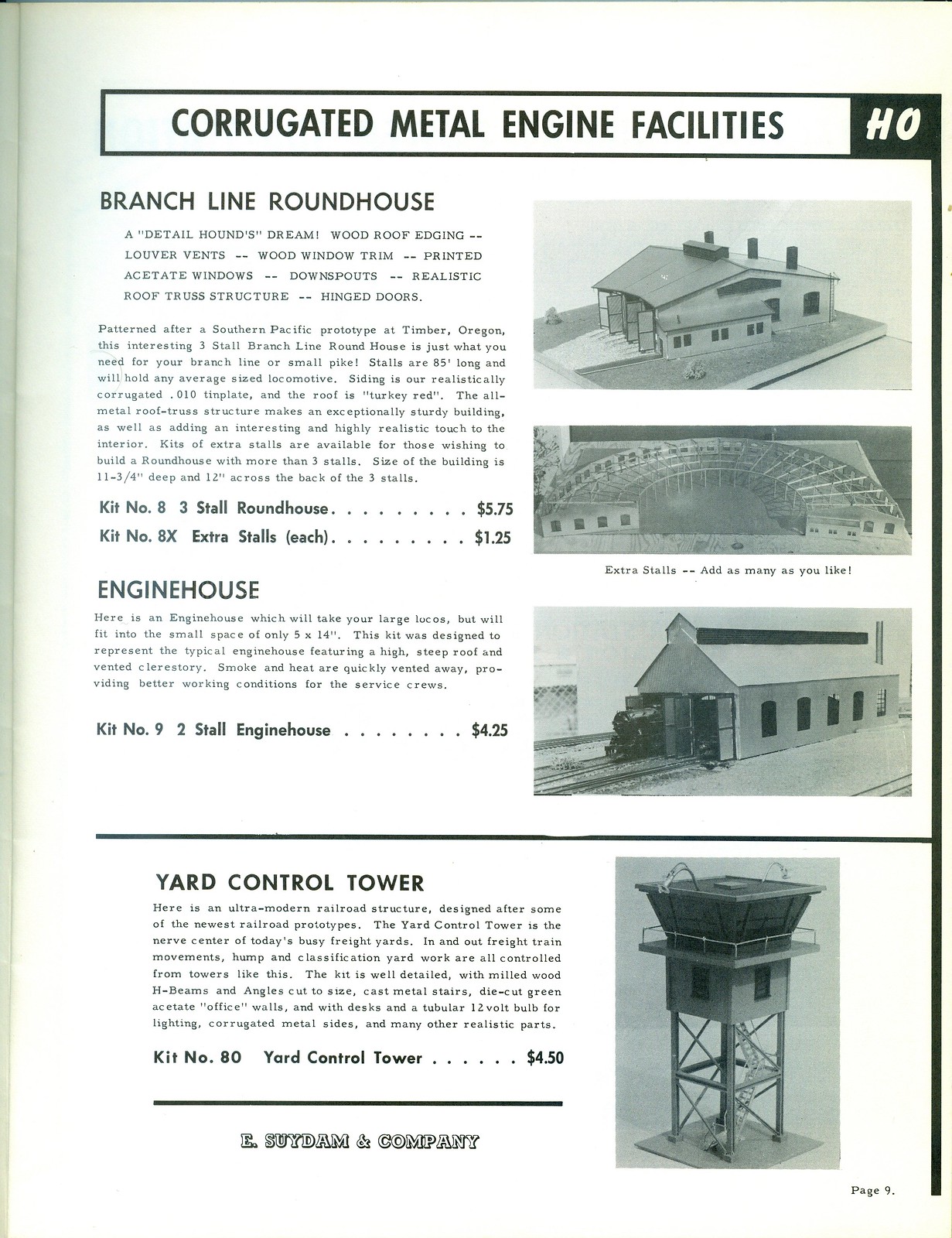The image is a detailed advertisement from a magazine or book, showcasing model kits for various train-related buildings and structures. It features a single sheet of paper that occupies the entire frame. Against a white background, there is extensive black text interspersed with images. 

The text across the top reads, "Corrugated Metal Engine Facilities," followed by "Branch Line Roundhouse, A Detail Hound's Dream, Wood Roof Edging." A detailed description explains that this model is patterned after a Southern Pacific prototype and outlines the various components like wood window trim, printed acetate windows, and a realistic roof truss structure. The roundhouse, which has three stalls to accommodate average-sized locomotives, measures 11 and 3/4 inches deep and 12 inches across, with additional stalls available for purchase. 

Another section describes an "Engine House," designed for larger locomotives, with dimensions of 5 by 14 inches. This kit features a high, steep roof and vented accelerator story for efficient heat and smoke dissipation. The text finishes with details about a "Yard Control Tower," another model kit available in the lineup.

On the right side of the sheet are four black-and-white photographs depicting the model structures: the Branch Line Roundhouse, Engine House, and Yard Control Tower. The images show detailed architectural features, emphasizing intricate designs suitable for model train enthusiasts. In summary, this advertisement presents a selection of highly detailed model kits for creating realistic train yard settings, with a strong focus on the quality and authenticity of the materials and designs.